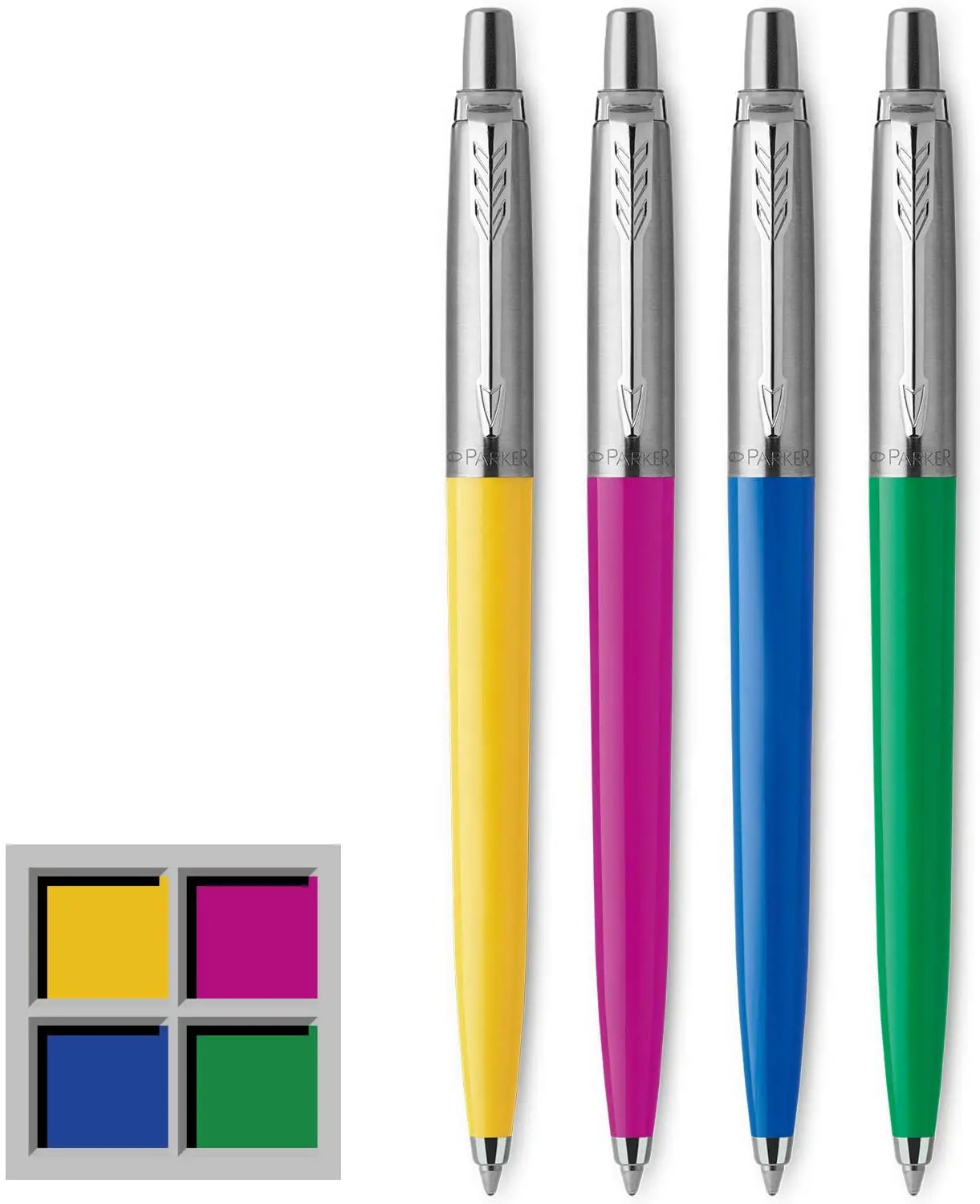This image showcases four click pens arranged in a row, each with a distinctive colored bottom: yellow, purple, blue, and green. The tops of the pens are silver, featuring ballpoint nibs also in silver, and a leaf design. To the left of the pens is a multi-framed square reminiscent of the old Microsoft logo, divided into four smaller squares each with a different color: yellow, pink, blue, and green. The overall background of the image is white, emphasizing the vibrant colors of the pens and the framed squares. The pens are brand new, and each pen's bottom half matches one of the four colors in the framed square arrangement.